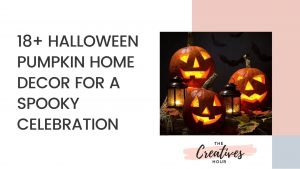This vibrant graphic showcases an enchanting Halloween-themed home decor setup, perfect for an 18+ spooky celebration. The image prominently features three large, round jack-o-lanterns with classic triangular eyes and noses, each uniquely styled mouth adding character to the trio. Accompanying the pumpkins are two ornate lanterns, each with six-sided glass panels and a rounded top adorned with a ring, casting an eerie glow from the tea candles inside. The caption clarifies the theme, indicating the decor is suitable for adults or features over 18 pieces. The name of the creative group behind this festive design, "The Creatives," is displayed, emphasizing their artistic contribution.